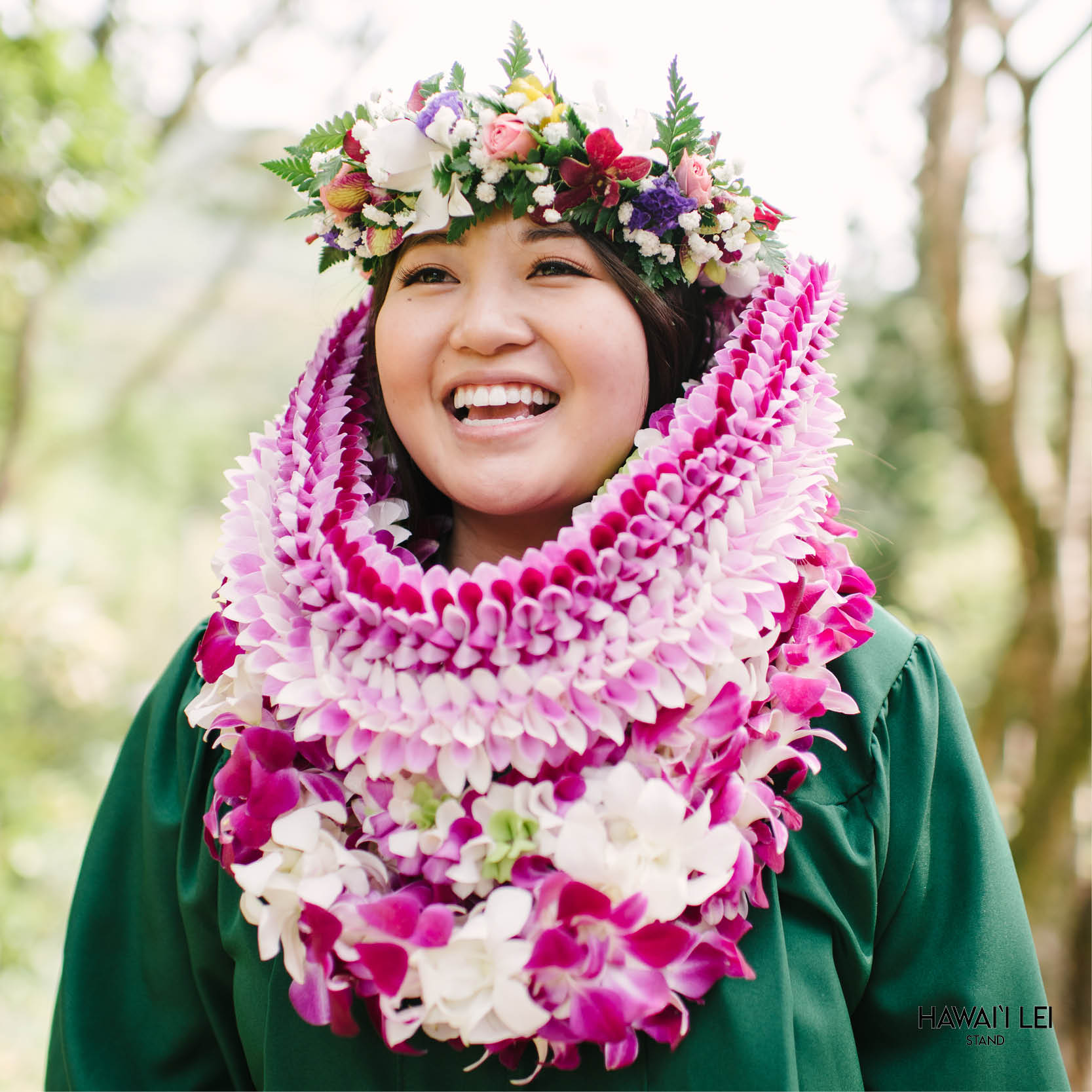The image depicts a joyful young woman, likely in her late teens to twenties, with dark hair mostly obscured by an elaborate floral headpiece. The headpiece is a vibrant mix of various colored flowers, including white, purple, pink, yellow, and red, intertwined with green leaves. She is beaming widely, revealing her teeth, and exudes happiness. Around her neck, she wears an ornate and thick U-shaped lei, composed primarily of red, white, and pink flowers, with a multitude of petals forming multiple layers. Below this main lei, another string of similarly colored flowers adorns her neck, cascading partially over a dark green robe. The background shows a hint of trees and vegetation, emphasizing the natural setting. The bottom right corner of the image reads "Hawaii Lay Stand," further suggesting a tropical locale and theme for the photo.